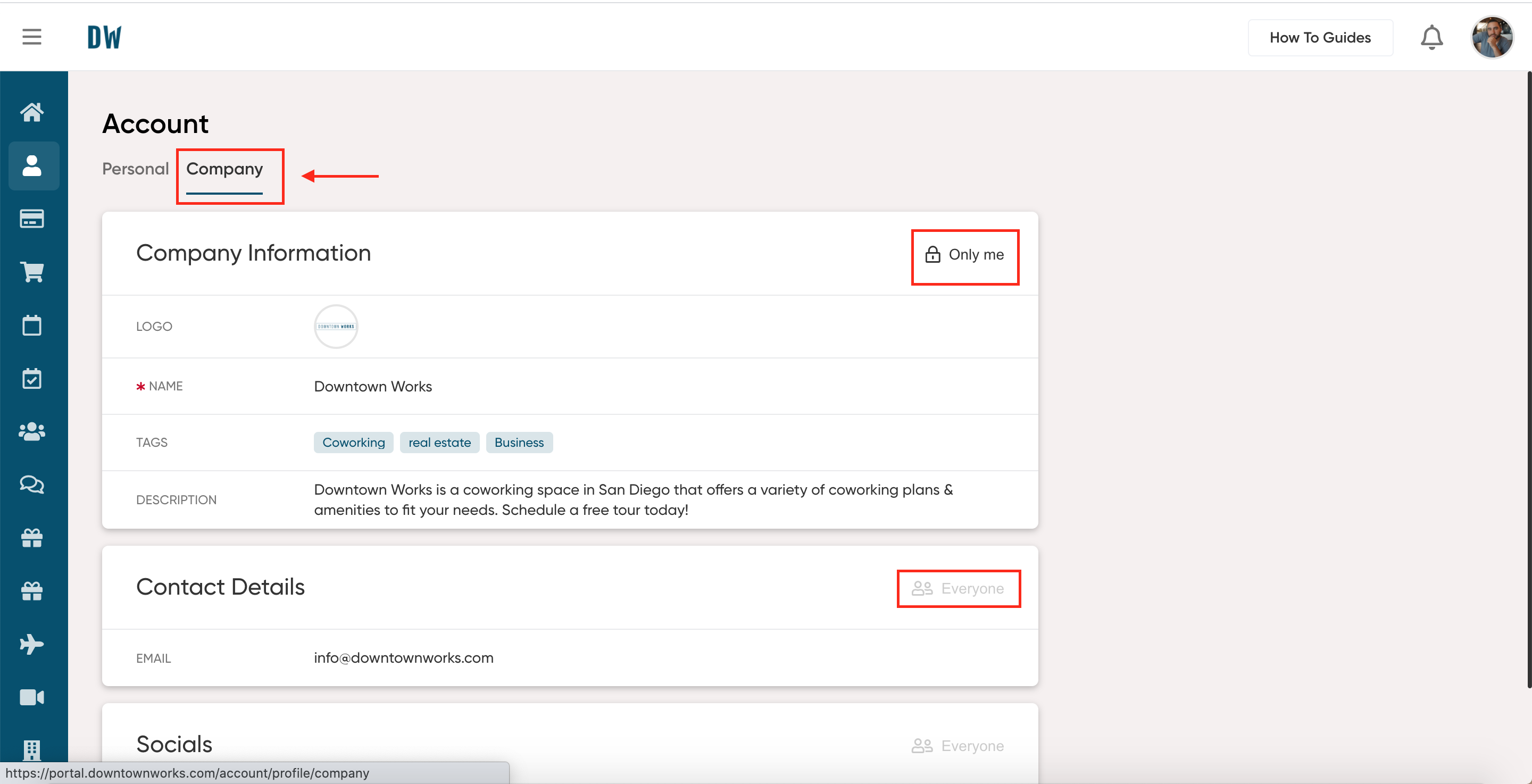**Webpage Detail Description:**

The image captures a detailed section of a webpage interface, starting with a very faint gray line at the top, beneath which lies a white border or band. On the left side of this band, there is a square consisting of three short stacked lines, likely representing the menu icon. Next to it are bold, teal, capital letters "D" and "W," presumably the user's initials. Moving to the right, there is a button labeled "How-To Guides," followed by a bell icon for alerts, and finally, a small, round profile photo, which is tiny and indistinct.

The background of the rest of the page is a very pale, purplish-gray color. Along the left side, there's a teal vertical bar containing a column of 13 white icons. This column appears scrollable as indicated by a thin black line on the right side of the page, suggesting you can click and drag to scroll down. The icons from top to bottom are a home icon, a user icon, a credit card icon (likely for payments), a shopping cart, a calendar, a calendar with a checkmark, a group of people, overlapping speech bubbles (likely for messages), a wrapped gift, another similar wrapped gift, an airplane, a video recording icon, and an unidentified icon that might be a domino or a calculator.

In the top left of the extensive purple-gray field, the word "Account" is displayed. Below this are two selectable options: "Personal" and "Company," with "Company" currently selected, highlighted with a red rectangular outline and a left-pointing red arrow. There are several white text boxes below this:

1. **Company Information:** Enclosed within a red rectangle is a padlock icon labeled "Only me." Details in this section include:
   - **Logo:** (Not visible)
   - **Name:** Downtown Works
   - **Tags:** Business, real estate, and an unreadable tag.
   - **Description:** "Downtown Works is a co-working space in San Diego that offers a variety of co-working plans and amenities to fit your needs. Schedule a free tour today!"

2. **Contact Details:** Includes the email "info@downtownworks.com" and a red-outlined rectangle on the right side saying "Everyone."

3. **Socials:** Appears empty or unreadable.

Finally, in the very bottom left, the URL is partially visible. It indicates a secure connection with "HTTPS" and includes segments like "portal/downtownworks.com/account" alongside some unreadable smaller text.

This comprehensive description articulates the layout and purpose of various elements within the webpage detail, providing a clear understanding of the interface for the viewer.